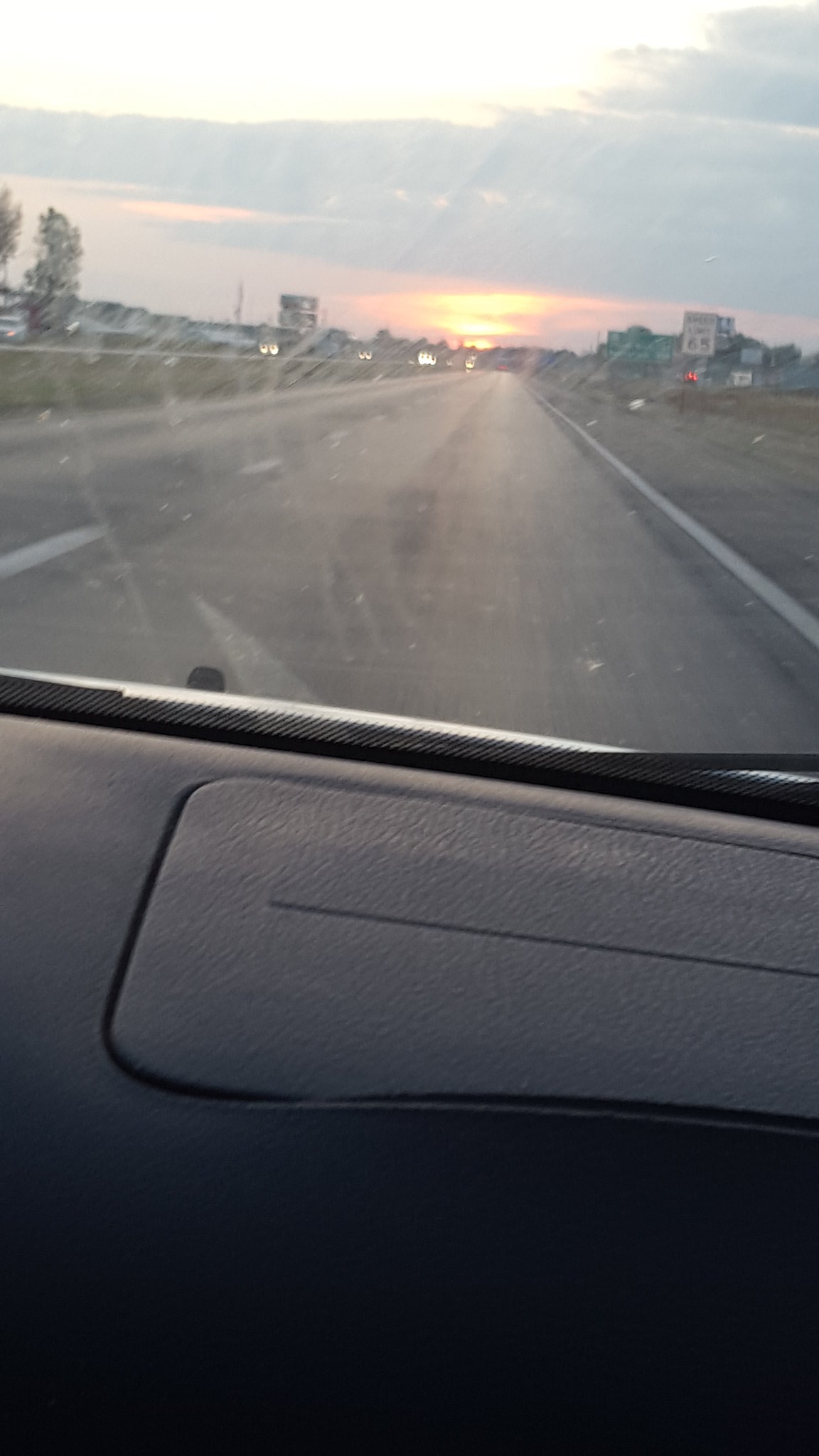This vertical image, resembling a still frame from a video, captures the perspective of a passenger seated in a car. The lower half of the picture reveals the car's dashboard, complete with the airbag compartment. In the upper half, the windshield opens up to a view of the highway ahead. The vehicle is cruising in the far right lane of a long, straight road.

Prominently visible outside the windshield are two road signs on the right. The first is a white speed limit sign indicating a maximum speed of 65 mph. Further ahead, though slightly out of focus, is a green highway sign likely pointing out upcoming exits or points of interest. The scene is bathed in the warm hues of the late-day sun, suggesting that it is nearing sunset.